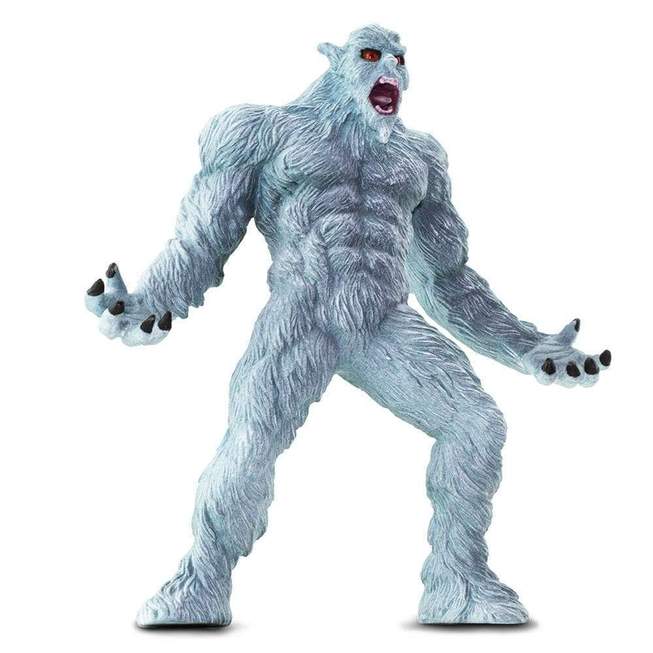This image shows a child's plastic toy depicting a cryptid creature reminiscent of both Bigfoot and the Abominable Snowman. The toy is primarily a mix of bluish, grayish, and turquoise hues, covered in light blue fur. The creature has a humanoid form with a muscular build, featuring pronounced six-pack abs on its chest. Its arms are extended outward, each hand equipped with five fingers ending in long black nails. The face of the creature is marked by its large, unnerving orange eyes with black pupils and an open mouth revealing sharp teeth on the top and bottom, as well as a reddish-black interior. It has pointed, curved-back ears and a very thick neck that appears wider than its head. The legs taper down to a widening at the base without distinct feet, resembling flat, rounded ends. The creature stands against a white background, leaning slightly to the left, evoking a sense of movement.